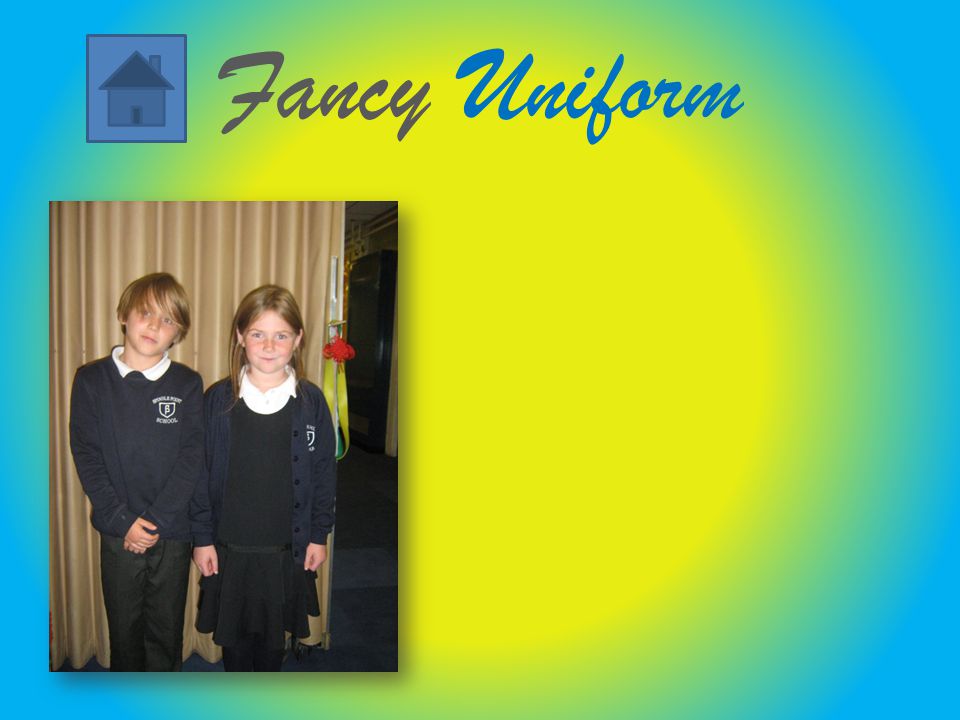This detailed image features a vibrant poster with a dynamic background, primarily composed of a large yellow circle, indicative of a sun, surrounded by a sky-blue expanse. The top section of the poster is marked by the text "Fancy Uniform," written in elegant cursive. "Fancy" is rendered in a grayish-purple hue, while "Uniform" is highlighted in bright blue. On the top left, encased within a small rectangular frame, there's a charming, cartoonish depiction of a house with a dark blue roof and a lighter blue body, set against a blue background.

Positioned on the left side of the image is a photograph capturing two Caucasian children who appear to be of a similar age, likely schoolmates. The child on the left is a young boy with black pants and a navy blue school shirt, covered by a black sweater, while the girl on the right wears a black dress complemented by black leggings and the same navy blue school shirt. They both don uniforms adorned with an indistinct emblem on the left side. Their blondish hair and poised appearance suggest a formal school setting, with a tan or beige curtain serving as the backdrop. This composition emphasizes the theme of school uniforms, encapsulated by the dual focus on the stylish text and the neat attire of the children.